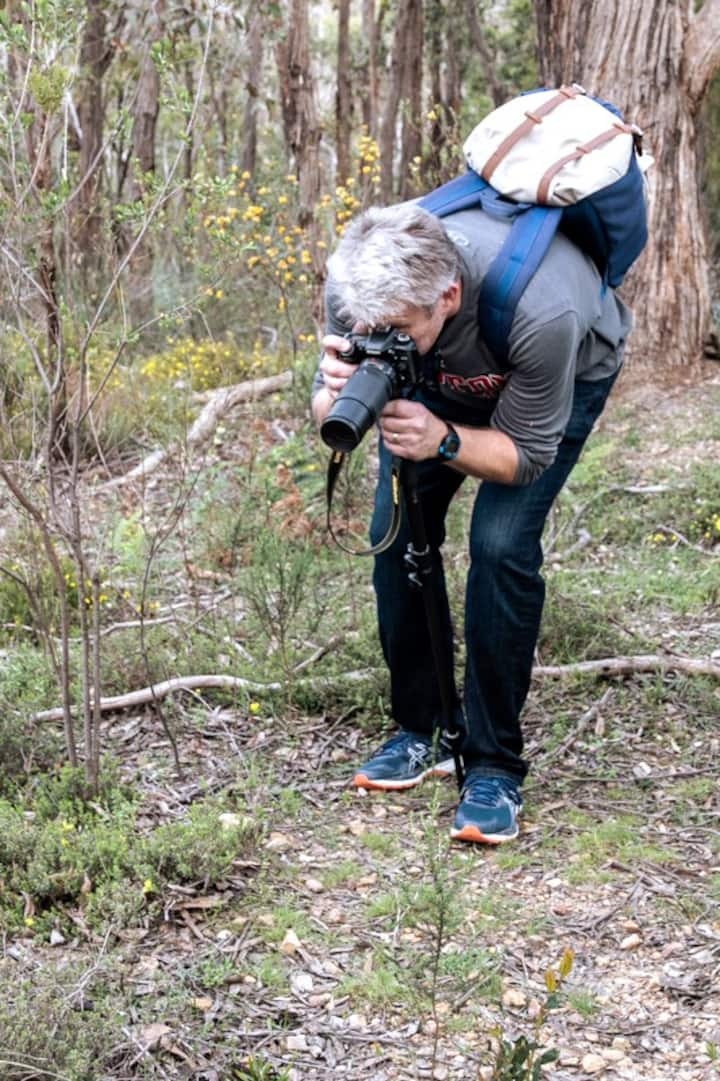In this vivid color photograph, an elderly man with gray hair is captured in the midst of a woodland area, focused intently on photographing something on the ground, likely vegetation or an unseen animal. He is slightly hunched over, holding a camera with a long telephoto lens close to his face, obscuring it from view. Dressed in a gray t-shirt, blue jeans, and blue tennis shoes, he also sports a blue backpack and has a wristwatch on his left arm. The wooded setting is detailed with numerous trees, some barren and others with foliage, with yellow flowers noted in the background. The forest floor is a mix of rocky terrain, grass, leaves, and small emerging plants. To his left, a small tree stands, while tree branches and additional ground vegetation add to the rich textures in the foreground.